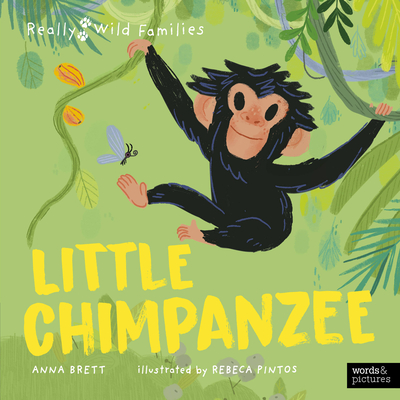The image is the cover of a children's book titled "Little Chimpanzee" in bold yellow text near the bottom. Below the title, in smaller white font, it reads "Anna Brett, illustrated by Rebecca Pintos." At the top left corner, the text "Wild Families" appears along with two paw prints in a hand-drawn style on a blue background. The central figure is a smiling, young chimpanzee with dark fur and white hand-like feet and hands. Its face is white with human-like features, including expressive eyes and white ears. The chimpanzee is swinging between two green vines, gripping one vine with its left hand. Surrounding the cheerful chimp are hand-drawn jungle elements, including a butterfly and various leaves and palm trees peeking in from the sides. In the bottom right corner, “Words and Pictures” is prominently displayed, indicating the book’s focus on young readers.